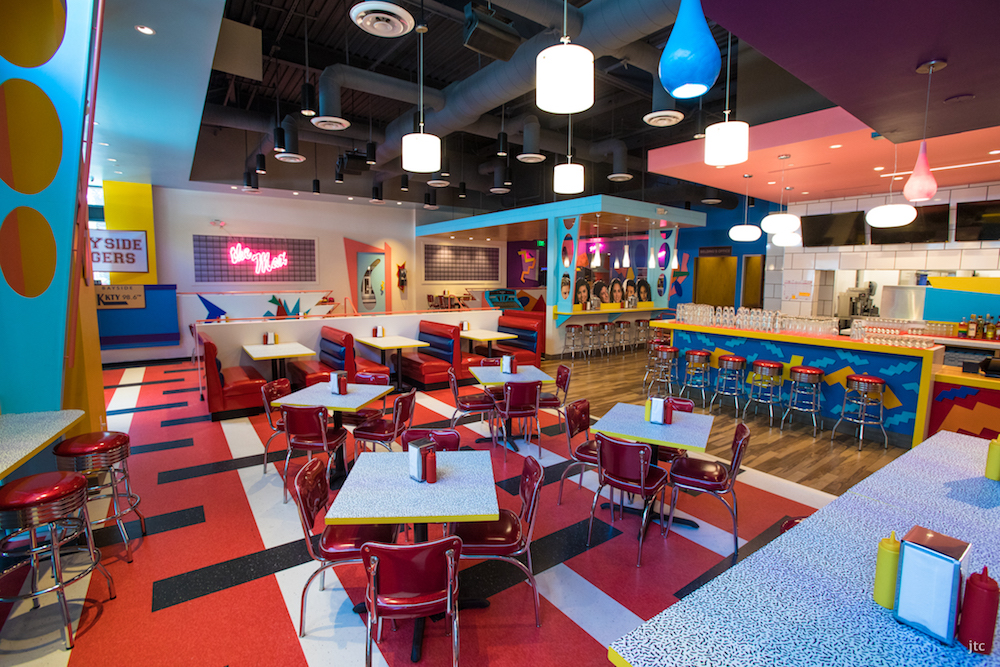This vibrant photograph captures the interior of a spacious, retro-styled dining area, possibly a school cafeteria or a themed restaurant, decorated with a blend of 1950s diner charm and 1980s colorful flair. The dynamic floor design features a striking red base with white longitudinal stripes and black crosswise dashed lines, contrasted by a section of brown wood plank flooring. Bright blue walls adorned with large yellow polka dots add to the festive ambiance. The tables, topped with Formica, are paired with shiny red patent leather, retro-style chairs, and complemented by chrome barstools with red seats along the bright yellow counter.

Pendant lights, both regular drum-shaped ones and bright blue glass ones, illuminate the space from the ceiling, which also features inset lights within coral-colored panels. The right side of the photo reveals a food prep or kitchen area, distinguished by a sleek counter where more barstools are arranged. The decor melds 1950s aesthetics with elements like squiggly blue and white graphics, as well as a hint of 1980s style seen in the neon signage and cardboard cutouts of faces. Although there are no people present, the room’s vivid colors and eclectic design make it a lively, engaging space perfect for socializing and dining.